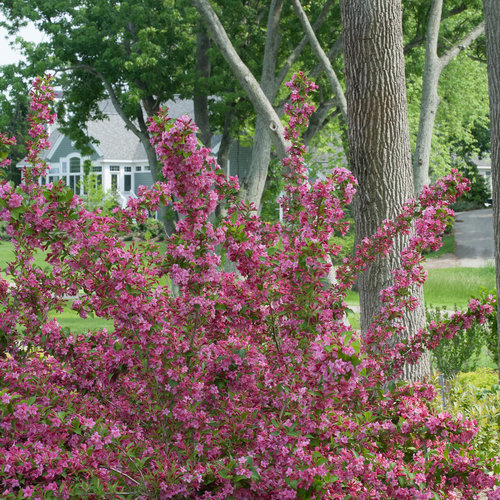The image showcases a vibrant, flowering shrub, lavishly adorned with tiny, bright pink flowers that densely cover its multiple extended stems. The shrub's lush green leaves and grass patches underneath add a refreshing contrast to the vivid pink blossoms, which dominate the scene. Behind the bustling bloom, a few trees stand with light green leaves, their trunks characterized by ripply, tan-brown and green bark. The background reveals a gray-roofed house with white trim, hinting at either a residential home or a clubhouse, possibly part of a country club. Additionally, a road extends to the right, suggesting the continuity of the neighborhood. A light blue sky glimpses through the treetops, enhancing the lively, springtime atmosphere, while light gray stepping stones meander through the composition, pointing towards the house and evoking a sense of serene, garden-like tranquility.